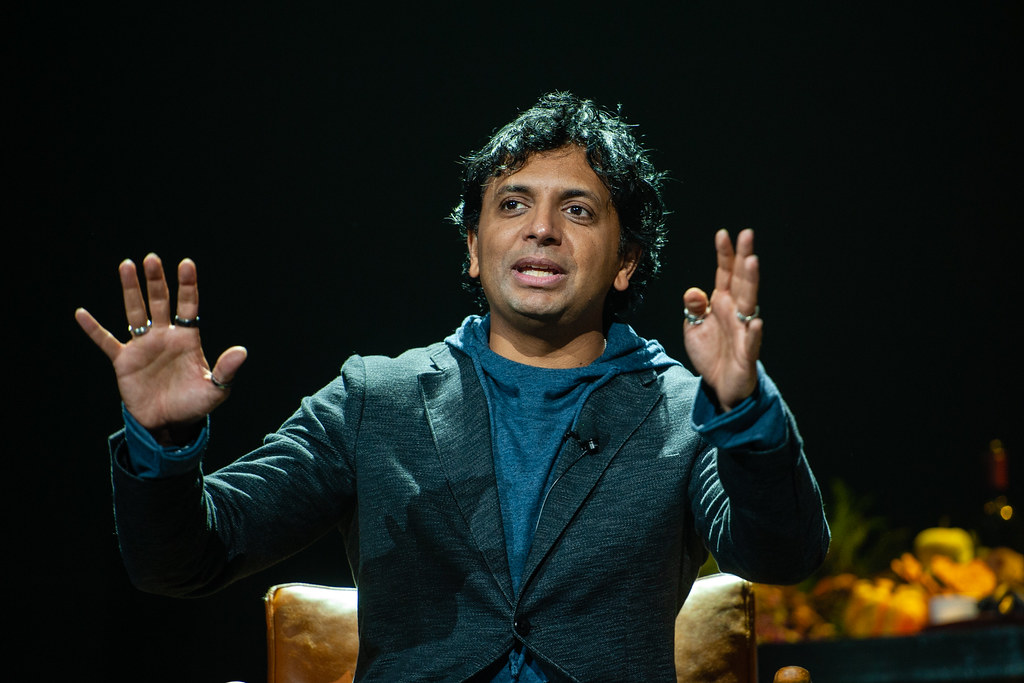In the photograph, a man with medium-length, wavy dark black hair and dark eyes is depicted gazing slightly to the left. He is captured from the stomach up, with both hands raised to shoulder height and open, displaying multiple rings on his fingers. His mouth is open, revealing both rows of teeth, suggesting he might be speaking or gesturing. The man is dressed in a greenish-colored suit jacket, buttoned just above the stomach, over a blue shirt. Additionally, a microphone is attached to his lapel.

The background of the image is primarily black, lending the scene a dramatic contrast, although there is a section on the lower right that is blurry but displays vibrant hues of green and yellow, possibly resembling food. The man appears to be seated on a brown, cushiony chair, visible at the bottom of the photograph.